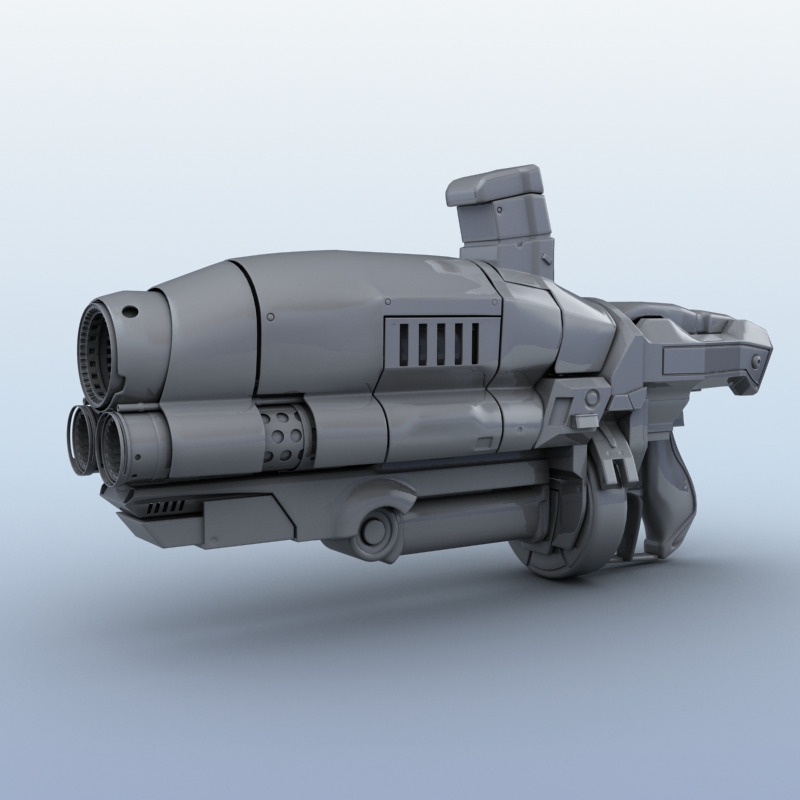This image showcases a highly detailed 3D rendering of a futuristic, sci-fi gun. The gun, portrayed in a shiny metallic gray, has a bulky and advanced design indicative of a weapon from an advanced future or a sci-fi adventure. It features three barrels, with a large central barrel flanked by two smaller ones. The gun points to the left, offering a three-fourths perspective. The model includes intricate details such as a circular tommy gun-style cartridge at the bottom, a modern-style cartridge protruding from the top, and five slats positioned at the front. Further detailing includes buttons, a trigger, and vents that suggest areas for emissions like bullets or plasma. The background transitions from a very light blue at the top to a dark gray at the bottom, and the gun casts a shadow on the ground below, enhancing its three-dimensional appearance. The rendering does not include any textures yet, leaving the gun’s surface smooth and reflective, and the overall scene possesses a clean, gradient backdrop, reinforcing the futuristic aesthetic.